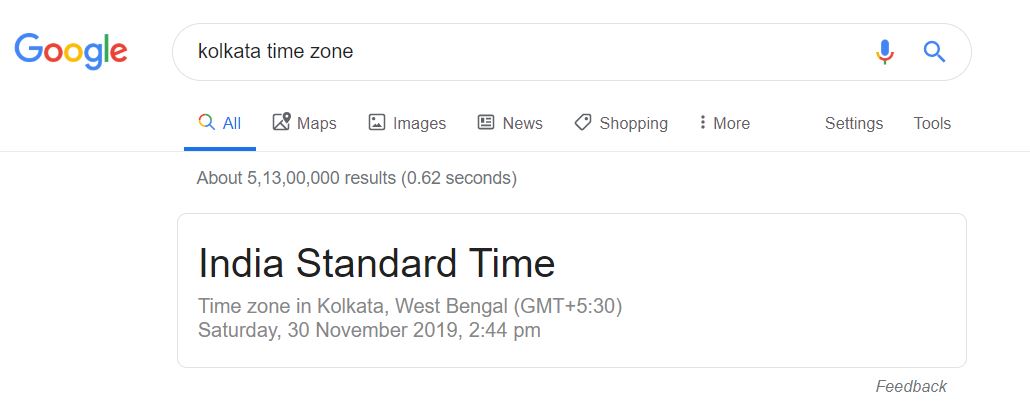This is a detailed screenshot from a Google web search with a white background. In the top left corner, the recognizable Google logo is displayed in vibrant colors: blue, red, yellow, blue, green, and red. Below the logo is the elongated, pill-shaped search bar where "Kwikata time zone" has been typed. The search bar also features a small microphone icon and a magnifying glass at the end.

Directly beneath the search bar are the standard Google search options menus: "All," "Maps," "Images," "News," "Shopping," and an additional button labeled "More," followed by "Settings" and "Tools."

Further down, the total number of search results is displayed, approximately five to six million, with the search executed in 0.52 seconds. The first result lists the time zone for Kwikata, West Bengal, indicating India Standard Time (GMT +5:30). The specific date and time provided in the result is Saturday, November 30, 2019, at 2:44 PM. At the bottom of the result, there is a discreet "Feedback" link.